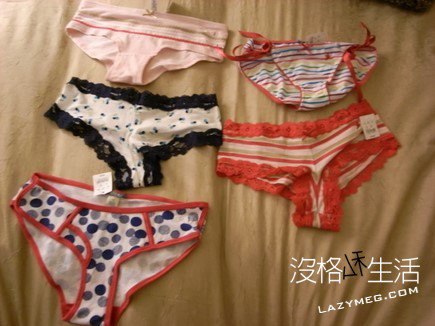The photograph features five pairs of women's or young girls' underwear carefully displayed on a golden beige, slightly wrinkled fabric background, likely for an online sale. The underwear is arranged in two rows: the top row has three pairs while the bottom row has two. The pair on the top left is pink and purple, and still has a price tag attached. To its right, a pair features a mix of white, red, yellow, and green. Below, the first pair on the left is white with red edges and gray and black dots, also with a price tag. Beside it, another pair is white with black borders and blue dots. The fifth pair, in the bottom left, is white with red edges and blue and light blue dots. At the lower right corner of the image is a mix of Chinese text followed by "lazymeg.com" in English.